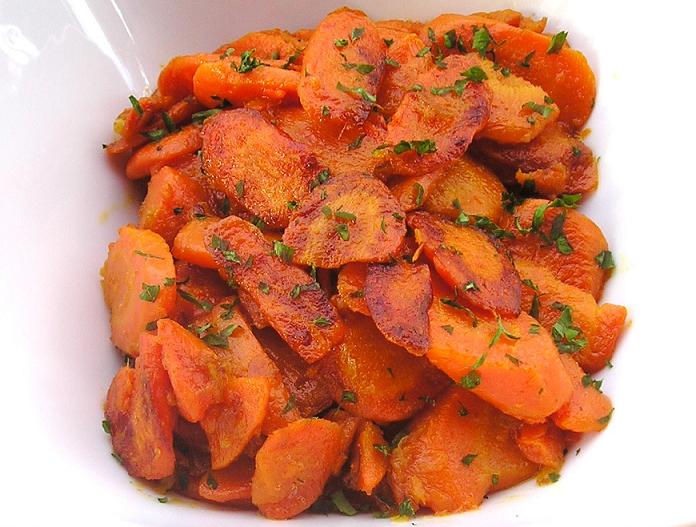The image displays a bowl of sizable, julienned carrot slices that have been expertly roasted to achieve a slight browning, especially concentrated on the top. The carrots exhibit a wet, juicy texture, suggesting they are well-cooked and tender, enough to crush easily between fingers. These vibrant orange pieces are notably seared, indicating they were likely pan-cooked or roasted, as evidenced by the dark patches on the edges. They are generously seasoned and sprinkled with fresh green herbs, which appear to be either parsley, cilantro, or green onions, adding a contrasting color and flavor. The presentation seems to be in a white porcelain dish, although the edges of the container are not visible, giving a top-down perspective of the neatly arranged and herb-topped carrots.